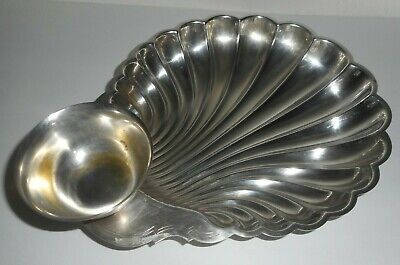This photograph captures a detailed, top-down view of a silver metallic utensil placed on a light gray background. On the left side of the utensil is a small silver bowl or cup, which is attached to a larger, intricate base. The base of the utensil is designed to resemble a peacock’s wings or a seashell, fanning out with sections that create a sense of movement and elegance. The reflective surface of the utensil catches light at various points, causing some areas to appear white while others maintain a darker, more traditional silver-gray hue. The craftsmanship highlights the varying textures and the reflective qualities of the metal, with the larger middle sections of the 'wings' or 'shell' being prominent and tapering off as they extend outward. The utensil lies empty, its design elements clearly visible against the consistent gray background, which provides a stark, yet complementary contrast to the shiny, silver utensil.